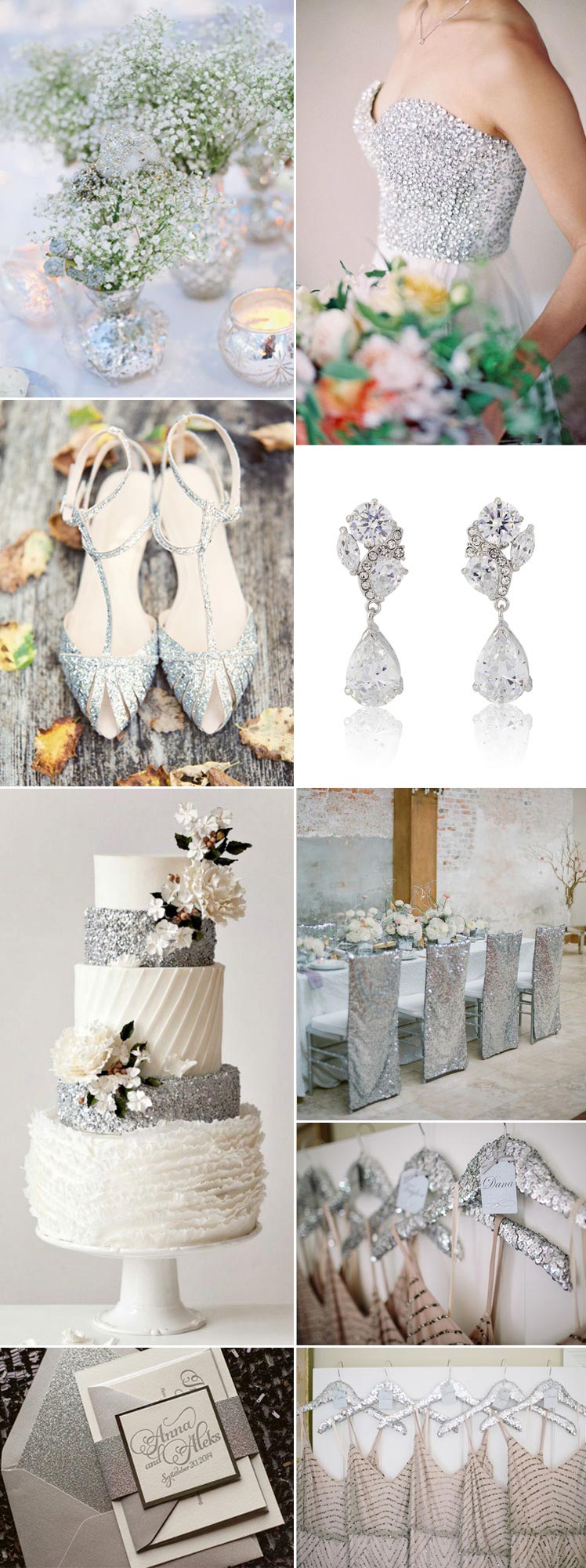This series of nine wedding-oriented photographs showcases various elements of bridal attire and accessories. Dominating the upper left corner are elegant white vases filled with delicate white flowers, likely intended for table decor. Adjacent to this, a stunning strapless gown embellished with sparkling jewels is displayed, accompanied by a vibrant bouquet of multicolored flowers. Moving right, a pair of intricately adorned silver T-strap sandals and a set of dazzling diamond earrings suggest bridal accessories. Center-left, a five-tiered wedding cake, exquisitely decorated in silver and cream, stands on a white table against an off-white backdrop. Below this, a formal dining setup, complemented by hanging bridesmaids' dresses in a closet, each labeled with names, adds a personal touch. The lower-left corner features an elegant wedding invitation, encapsulating the event's tone. The entire composition weaves together the meticulous details and preparation that encapsulate a wedding celebration.